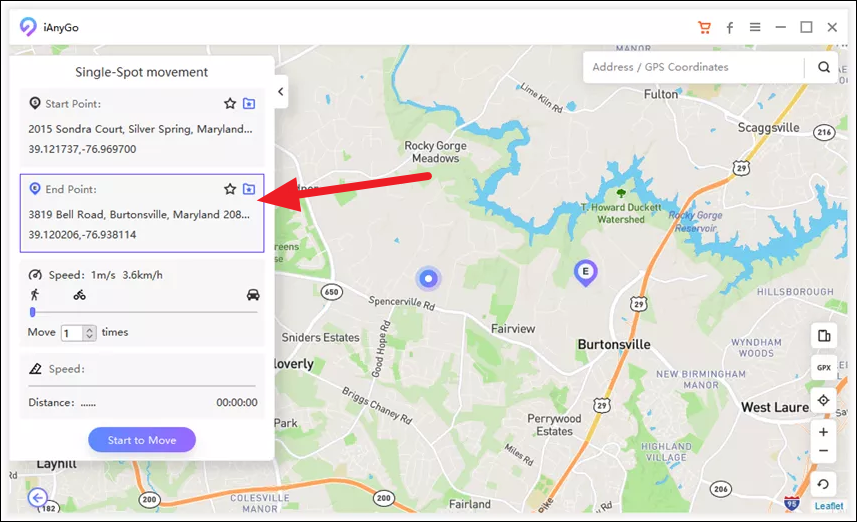A detailed caption for the image described:

The image showcases a website interface primarily featuring a digital map as the background. At the very top, there is a navigation bar with an icon followed by the text "INEGO," a small shopping icon on the right, an "F," three horizontal bars, a box, and an "X" symbol. Towards the top right corner of the page, there's a search bar labeled "Address" for GPS coordinates.

On the left side of the webpage, there are distinct input boxes with a white background and light gray individual sections. The first box is labeled "Start Point" and contains the address "2015 Sundercourt, Silver Spring, Maryland" with the coordinates "39.121737, -76.969700." Below it, the "End Point" is listed as "3819 Bell Road, Burtonsville, Maryland" with the coordinates "39.120206, -76.938114," indicated by a red arrow and enclosed in a purple square border.

The third section provides movement options and is divided into sub-categories featuring a person, a bicycle, and a car symbol on the right, labeled "Speed" with options of "1m/s" and "3.6 km/h." A dropdown menu allows the user to select movement intervals with "1" being one option, alongside a label marked "times."

The fourth and final section displays "Speed Distance" in a digital timer format "00:00:00" with a "Start to Move" button below it. Bold text at the bottom of the image states "Burtonsville and West Laurel."